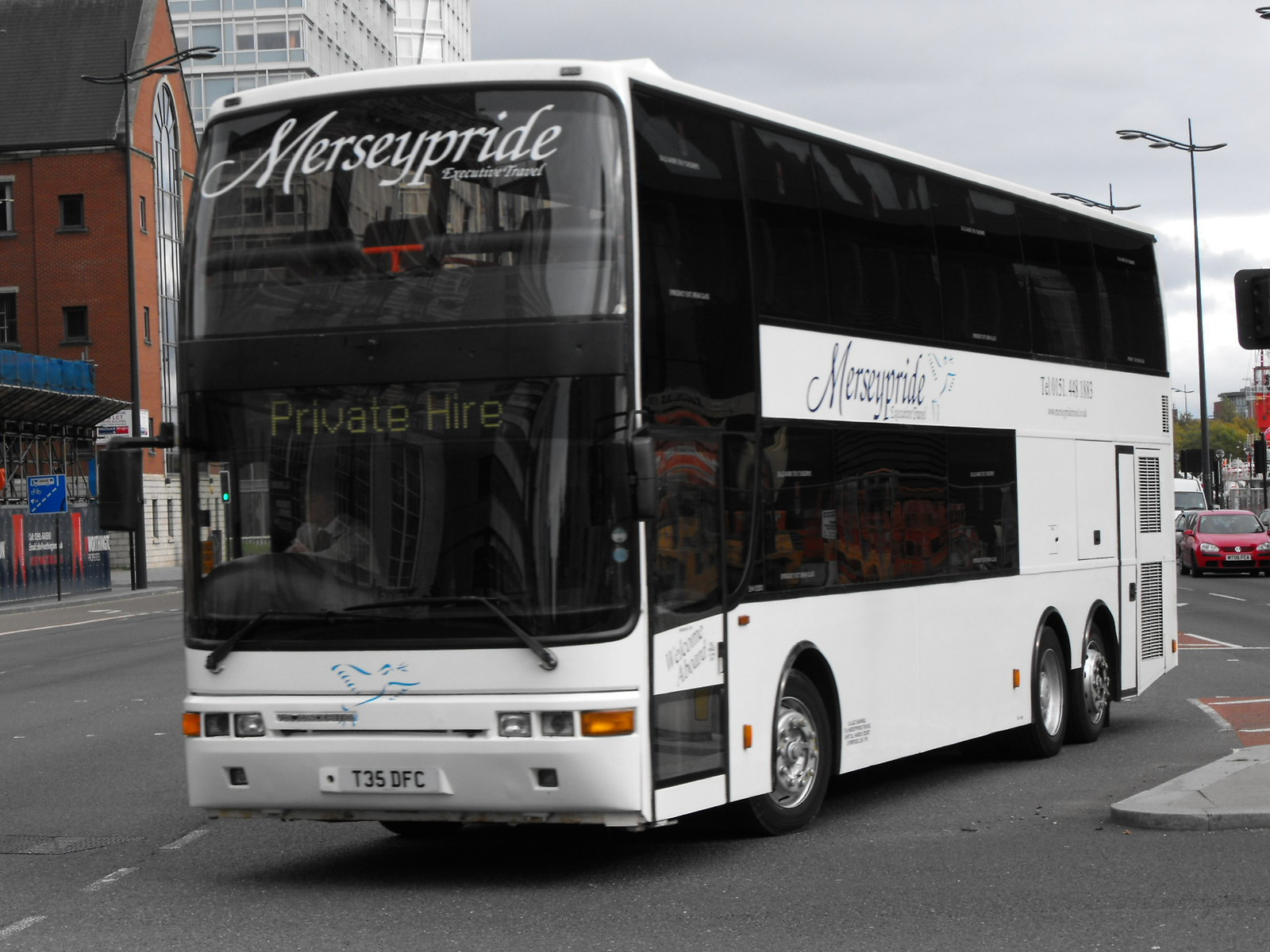In this detailed image, we see a large, clean, and well-maintained white double-decker bus prominently positioned on a city street. The bus, belonging to the company Mercy Pride Executive Travel, features the company's name, "Mercy Pride," prominently displayed at the top front, along with "Executive Travel." Below these, the sign reads "Private Hire," indicating the bus is available for rent for transportation and events. Its windows are blacked out, enhancing its sleek appearance. The detailed license plate number on the front of the bus is T35 DFC. Inside, behind the windshield, the driver is visible, dressed in a white shirt and black tie uniform.

Surrounding the bus, the cityscape includes a brown building with a gray roof on the left side of the picture, adding to the urban backdrop. Directly behind the bus is a red car, also positioned on the street, with its license plate clearly visible. Additional vehicles can be seen, suggesting moderate traffic. The sky overhead is overcast, setting a muted tone for the scene. The overall atmosphere portrays a typical day in the city, with the bus making a right turn amidst the surrounding architecture and vehicular activity.